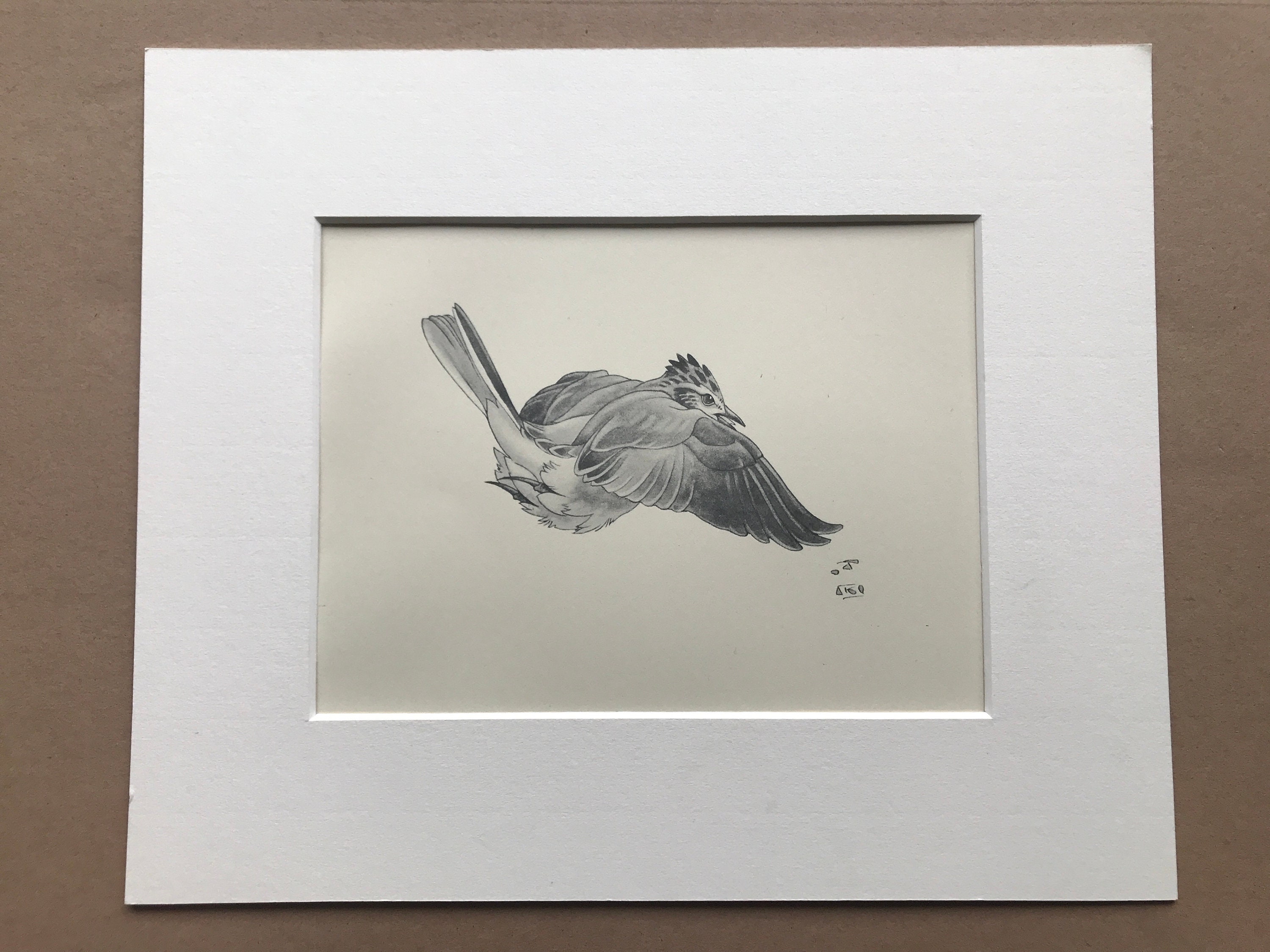The image presents a detailed charcoal pencil drawing of a bird in flight, centered within a thick, white frame. The bird, characterized by its short, round body and medium-length tail, is depicted facing to the right with its right wing fully extended. Intriguingly, its legs appear to be extended behind it, adding a unique perspective to the composition. The drawing features intricate shading, particularly on the wings, demonstrating the darker hues characteristic of such a bird, possibly a jay or ground-foraging bird due to its long, pointed beak. The feathers at the bird's neck form a crown-like pattern, adding to its majestic appearance. In the bottom right corner of the drawing, small, unreadable scribbles can be seen, likely the artist's signature. The framed artwork is set against a plain brown surface, enhancing its monochromatic aesthetic.